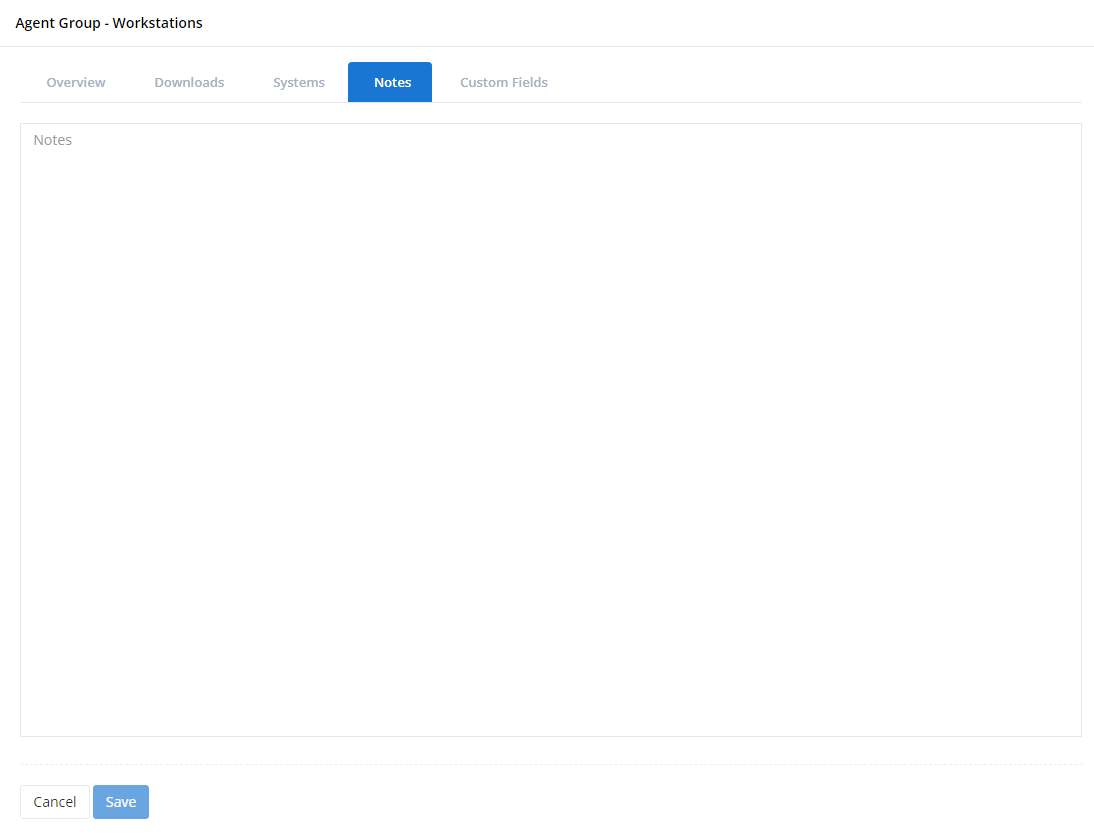The image displays a web interface with a clean, white background. In the top-left corner, the title "Agent Group-Workstations" is prominently featured in black font, with the first letter of each word capitalized. Directly beneath this title, a gray line spans the width of the page, delineating the title from the menu options below it. 

The menu options, listed from left to right in light gray font, include: "Overview," "Downloads," "Systems," "Notes," and "Custom Fields." Among these, the "Notes" option is highlighted with a blue box, indicating that it is the currently selected section. A second gray line runs horizontally beneath the menu options, further sectioning off the page. 

Dominating the main content area is a large gray box. In the top-left corner of this box, the word "Notes" is displayed, signifying that the user is in the notes section and has the capability to write a note. This area is an empty text box with a gray outline.

At the bottom-left of this text box, there are two buttons for user actions. The "Cancel" button is white with black text, while the "Save" button is blue with white text. Both buttons provide options to either discard or save the entered note, respectively. 

The overall layout is simple and uncluttered, with a consistent white background throughout the interface.